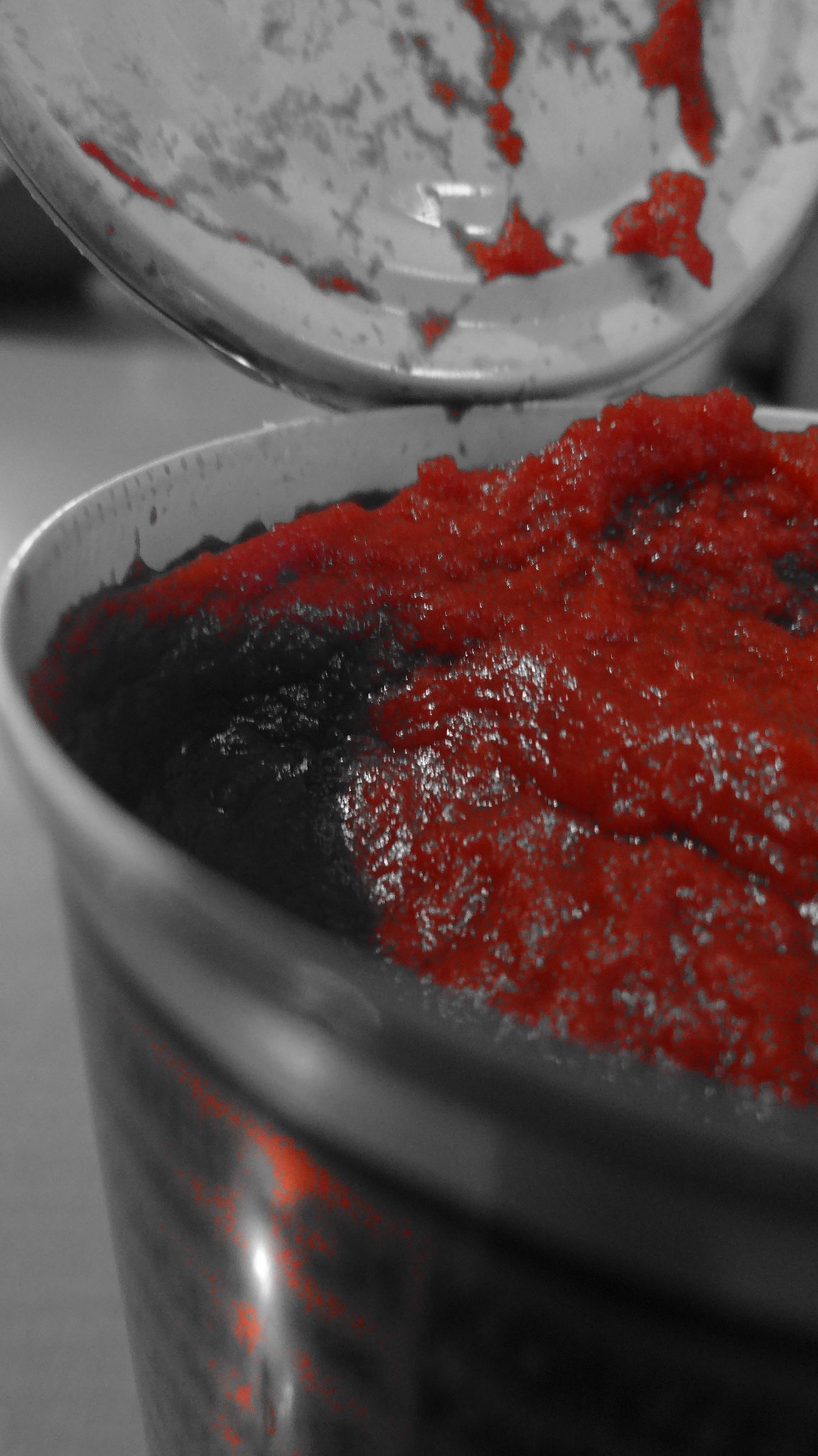The photograph showcases a clear plastic Tupperware container filled with a thick, bright red, and creamy substance. The container has an equally clear lid that is partially removed and held up, revealing some of the red substance adhered to it. The image is poorly lit, with a dark upper background fading into a blurry, plain white lower background. The container appears almost full, with the vibrant red content resembling either pureed beets or a similar sauce. The outer part of the container features a red label with black letters, although the label details are not the focus. Some areas of the red substance look slightly burnt or discolored. The overall scene is tightly zoomed in, emphasizing the container and its contents against an otherwise nondescript white background.